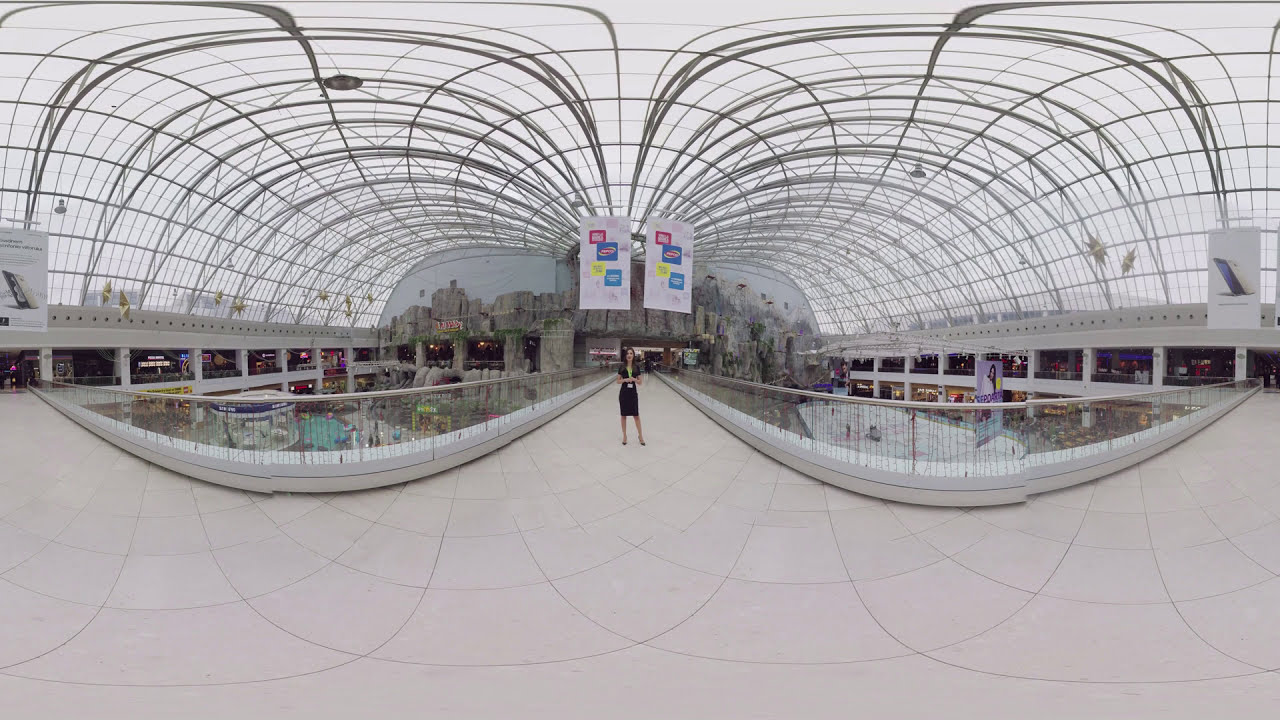This photograph captures the interior of what appears to be a bustling, multi-level shopping mall with a distinctive architectural design. Central to the image is a young woman in a sleek black dress and high heels, standing in the middle of a cream-colored, intricately tiled walkway. Her hands are clasped in front of her, and she stands poised, somewhat distant from the camera. The mall's ceiling is a striking feature, composed of spiraled, arched metal bars forming a transparent roof, which reveals a gray sky above and gives the space a greenhouse-like ambiance. 

Behind the woman are metallic railings separating the first-floor walkway from the ground floor below, which is teeming with people. To her left and right, curved railings delineate the edges of the aisle, and rectangular shop windows showcase various activities, reinforcing the mall's lively atmosphere. Additionally, a conspicuous advertisement poster is visible in the background, adding to the commercial setting. The overall scene is vibrant and dynamic, filled with the energy of shoppers and the unique aesthetic of the mall’s modern design.